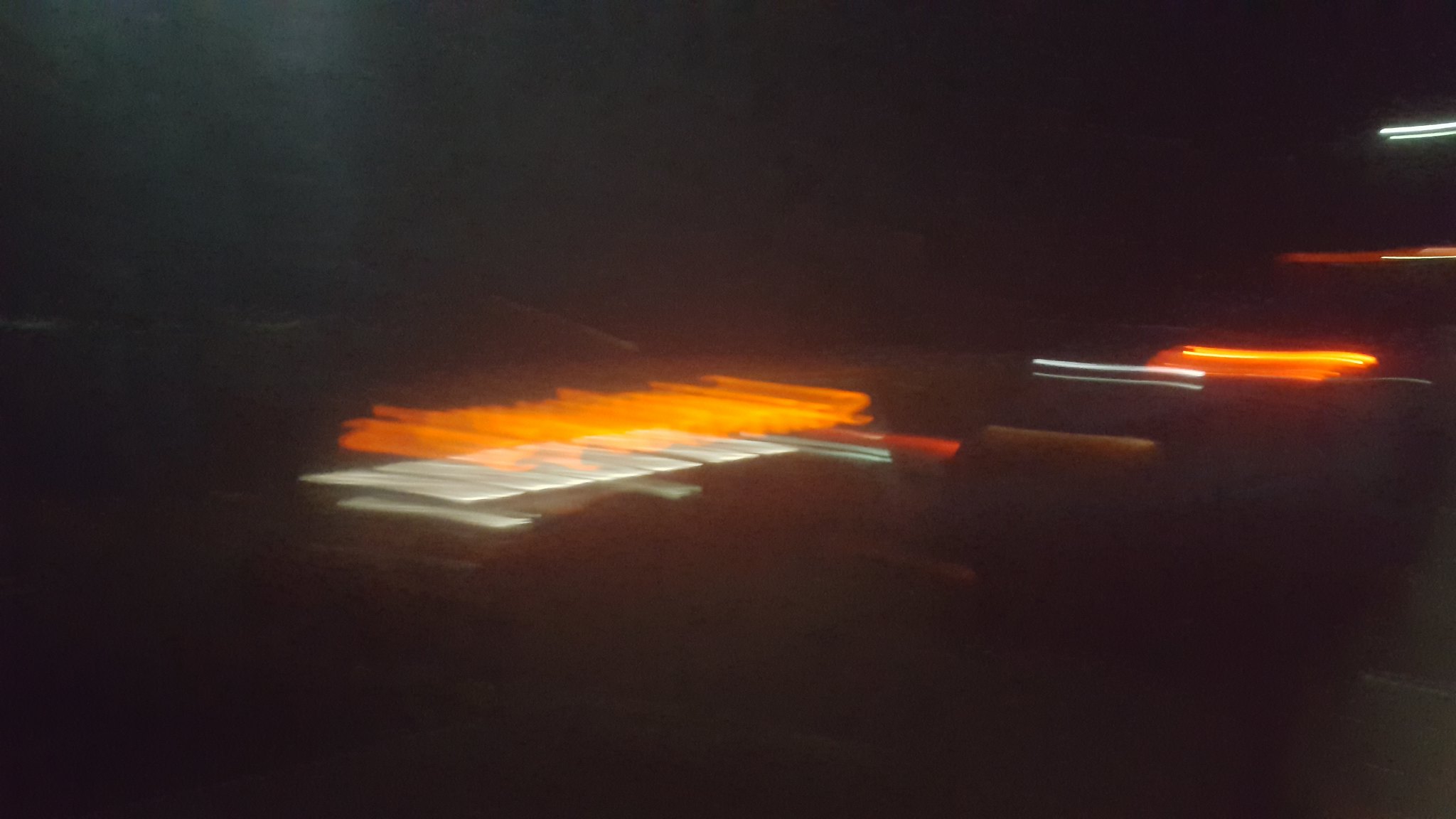The image is a very blurry nighttime shot predominantly featuring streaks of light. The lights are mostly orange and red, possibly from vehicle headlights or neon signs, creating horizontal, zippy, and squiggly patterns against a largely black background. The blurry streaks, extending up to five times their original size, suggest a slow shutter speed capturing the scene possibly from a moving car. In the foreground, what appears to be the back of a neon sign is partially legible, with a backward 'S' and possibly other letters like 'A' or 'I' trailing off. There are additional scattered lights, ranging from white to reddish, positioned in a more or less horizontal line. The top left of the image has a grayish area, while the rest of the colors blend into a hazy mix of gray, reddish, brownish, and black, indicating a poor-quality capture. The overall scene is devoid of much vertical structure, with most elements extending laterally across the frame.